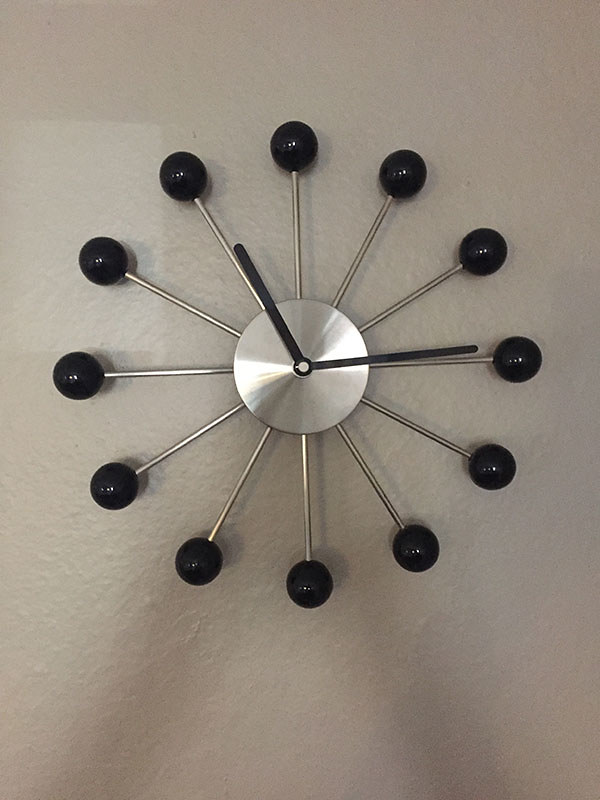This image showcases a mid-century modern wall clock, elegantly mounted on a gray-painted drywall. The slightly textured surface of the drywall adds subtle depth to the backdrop. The clock itself features a minimalist design, with a small, polished silver circle at its center. Radiating outward from this center are twelve sleek silver spokes, each tipped with a black ball, effectively marking each hour. Both the hour and minute hands are also black, providing a striking contrast to the stainless steel silver hue of the clock’s structure. This sophisticated timepiece not only tells time but serves as a stylish focal point on the understated gray wall.